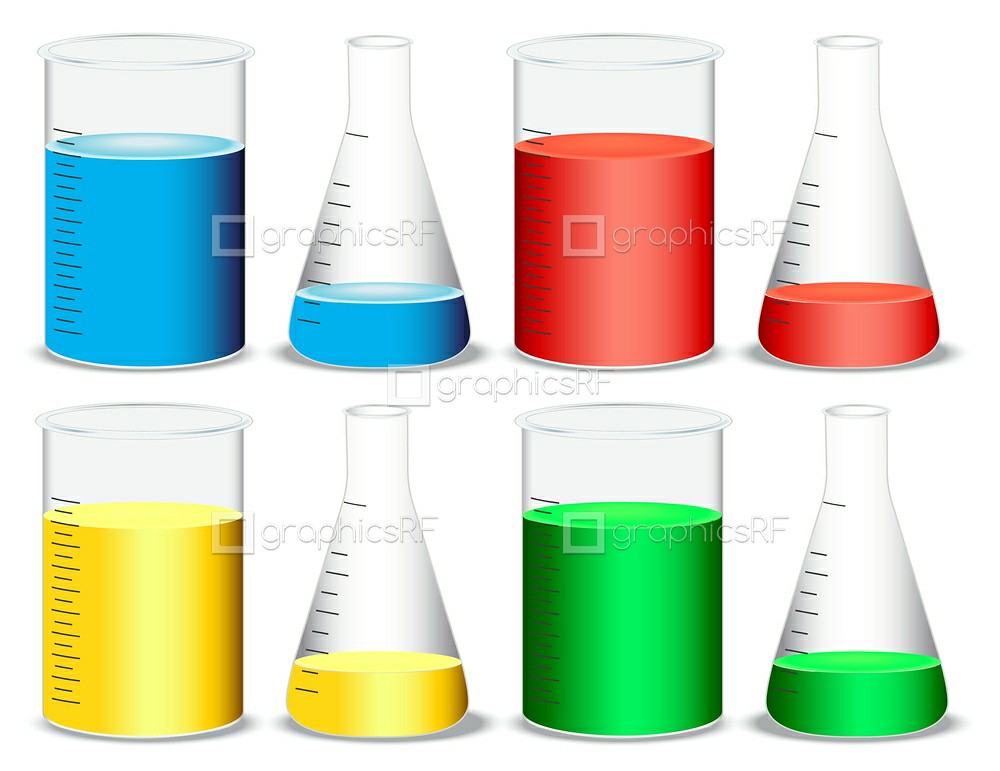This stock image is a detailed infographic of various scientific beakers, precisely drawn, likely by computer, illustrating their stereotypical forms. The image features eight beakers split into two rows, with each row containing a pair of cylindrical and a pair of conical (or triangular) beakers. Each beaker is filled with colored liquid: blue, red, yellow, and green, distributed such that each color has both a cylindrical and conical beaker counterpart.

In the top row, the blue cylindrical beaker and the blue conical beaker are filled approximately three-quarters high, while the adjacent red cylindrical and conical beakers are filled to the same level. Similarly, in the bottom row, the yellow cylindrical and conical beakers are also filled to three-quarters, as are the green cylindrical and conical beakers. Notably, the cylindrical beakers consistently hold more liquid compared to their conical counterparts, which are filled to about one-sixth.

The background prominently displays the "Graphics RF" watermark, a square logo that appears repeatedly across the image in five places, ensuring brand visibility. The detailed design, including perfect dashed lines on the beakers, further emphasizes the precision of this computer-generated drawing. The text near the logo is barely visible but present, contributing to the image's polished and professional appearance.